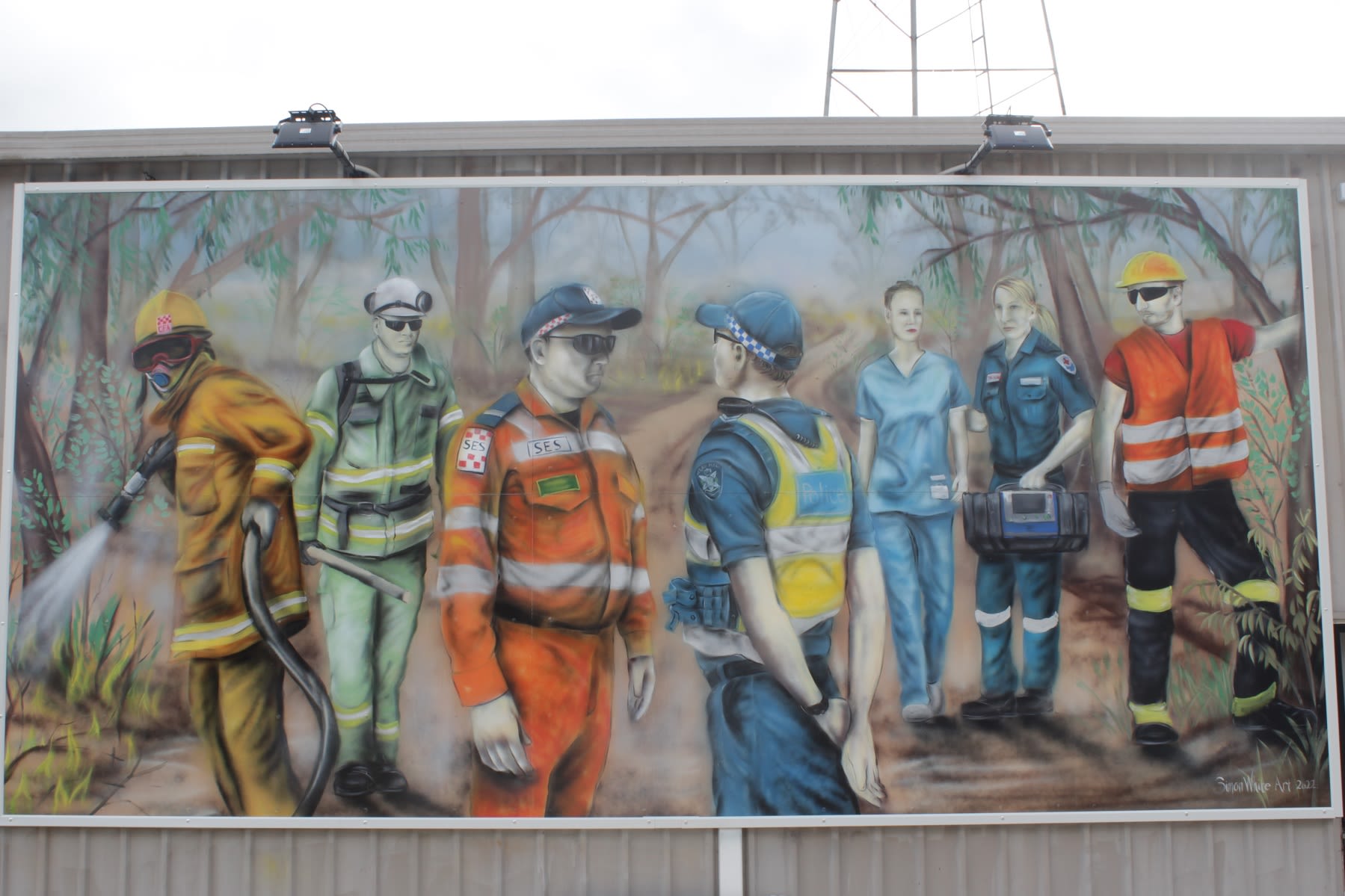The photograph captures a detailed hand-painted mural displayed prominently on a billboard or the side of a building with gray walls and a visible antenna tower in the skyline behind it. The mural, featuring a forest background with trees and a dirt path, depicts a group of seven first responders and service workers standing together in a unified and serious stance. From left to right, the figures include:

1. A firefighter dressed in a yellow outfit, actively spraying water, likely targeting a forest fire.
2. A forest ranger or similar role, positioned next to the firefighter and dressed in green.
3. A police officer in a blue uniform with a yellow vest.
4. A rescue squad member or another first responder in an orange outfit.
5. Two healthcare professionals – a nurse and an EMT, both wearing blue uniforms.
6. A construction worker at the far right end, identifiable by his construction hat and sunglasses.

The mural portrays these workers in collaborative action within a dimly lit, forest-like setting, emphasizing their roles and cooperation in handling emergency situations. The absence of text draws attention solely to the depicted scene and the characters' professionalism and dedication.